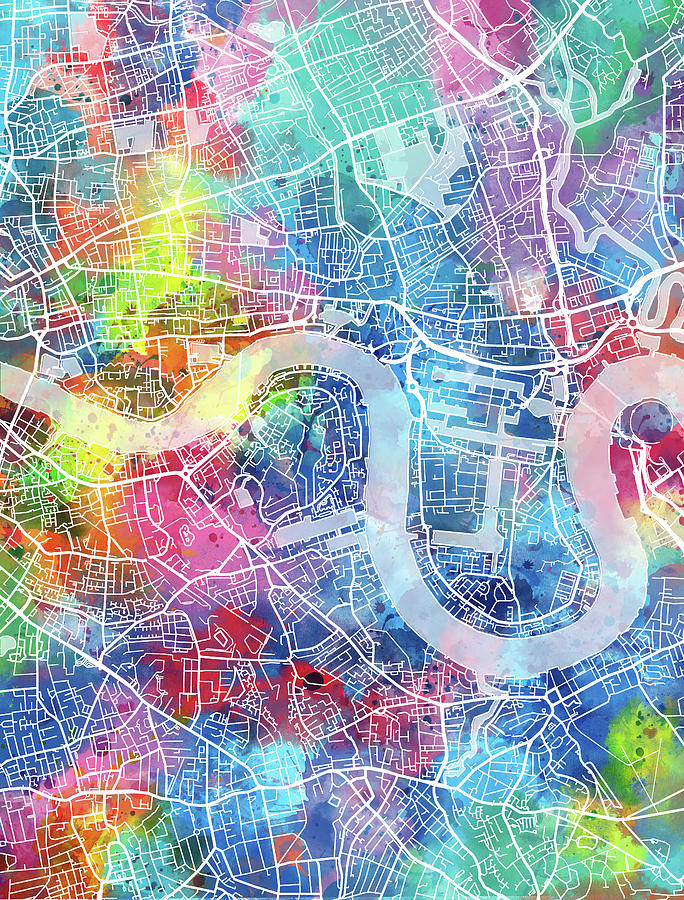The image depicts a vibrant, cartoony map of a city from a bird's-eye view. Central to the image is a winding river, represented by a semi-transparent, thick line that snakes horizontally from left to right. The city's layout is detailed with white lines indicating various streets, from thick highways to thin residential roads. The land areas between these streets are filled with a kaleidoscope of tie-dye colors—yellows, oranges, purples, blues, teals, pinks, reds—that bleed into one another like watercolor, creating a cloudy, yet harmonious backdrop. The entire image resembles a poster with an artistic, multicolored representation of the city's street outlines against a dreamy, abstract landscape.